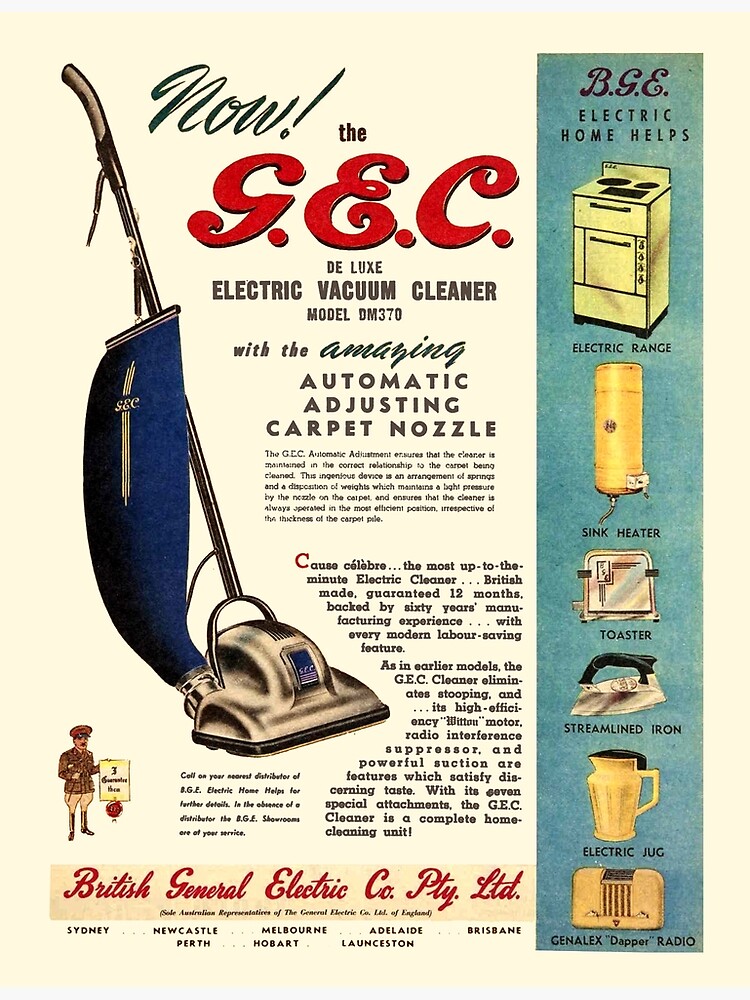The image is a vintage advertisement for the GEC Deluxe Electric Vacuum Cleaner, model DM370, featuring the revolutionary automatic adjusting carpet nozzle. The layout is in portrait orientation, primarily in black and white, with touches of blue, green, and yellow for emphasis. Dominating the left half of the page is an illustration of the upright vacuum cleaner with a blue bag attachment. To the right, a vertical blue panel titled "BGE Electric Home Helps" showcases six illustrations of home appliances: an electric range, sink heater, toaster, streamlined iron, electric jug, and a Genelec Dapper radio, each labeled in black text.

At the top, the headline reads in a mix of black and red, "Now! the GEC Deluxe Electric Vacuum Cleaner Model DM370 with the amazing automatic adjusting carpet nozzle." A drawing of the vacuum cleaner is accompanied by several lines of descriptive text in a foreign language, detailing the product's unique features.

In the lower left corner, there is a detailed line art illustration of a man in a brown uniform. At the bottom of the page, a band in dark cream color with bold red text announces "British General Electric Co. Pty. Ltd." with additional location details in black beneath it. The entire design exudes an old-school charm, typical of mid-20th-century print publications.